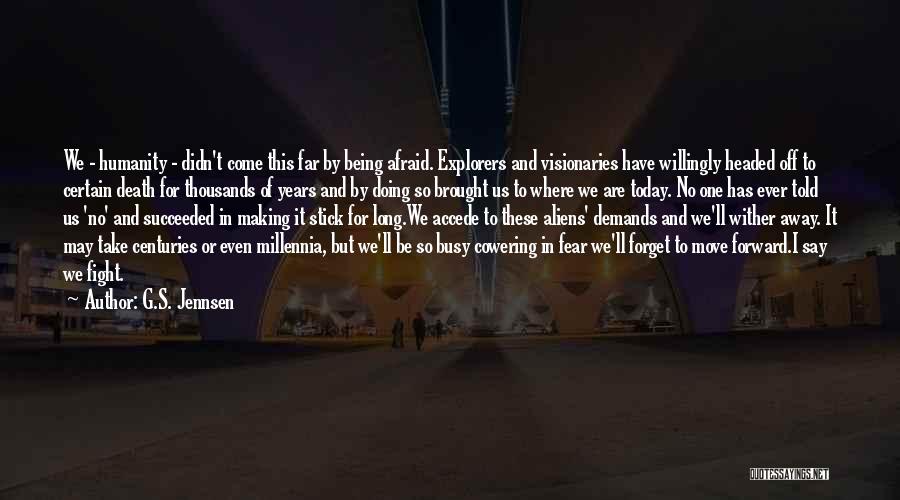The image features a dark, somewhat blurry photograph of a futuristic cityscape with scattered lights, buildings, and people standing on what appears to be a grey pavement between elevated structures resembling subway tracks. In the background, the urban environment fades into the distance, adding depth to the scene. Superimposed prominently in the center is a large paragraph of white text, which reads:

"We, humanity, didn't come this far by being afraid. Scholars, explorers, and visionaries have willingly headed off to certain death for thousands of years, and by doing so, brought us to where we are today. No one has ever told us no, and succeeded in making it stick for long. We accede to these alien demands and we'll wither. It may take centuries or even millennia, but we'll be so busy cowering in fear that we'll forget to move forward. I say we fight." 

This powerful quote by author G.S. Jensen stands out starkly against the dark backdrop. The image, with its combination of text and a futuristic urban setting, evokes a sense of determination and defiance against overwhelming odds.